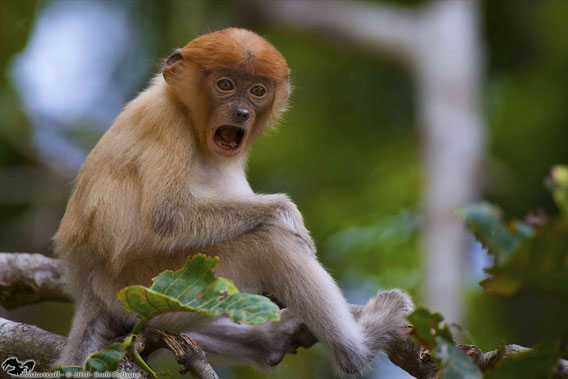This color photograph captures a detailed close-up of a smaller species of monkey in an outdoor, natural setting. The monkey, which features a striking reddish fur atop its head and a predominantly tan and gray body, is perched on a fig tree branch. Its body is positioned with the back toward the left side of the image and the belly facing the right, while it turns its head dramatically to the camera with a wide-open mouth, revealing its teeth and tongue in what appears to be a scream or a vocalization. The monkey's brown eyes are wide open, adding to its expressive appearance. Its right arm rests on its knee, and both its legs and a part of its tail are visible, gripping the branch for balance. The background of the photograph is blurred, filled with indistinct greenery and tree trunks, emphasizing the focus on the monkey. Scattered across the branch are a few green leaves, some of which have been chewed on by insects, enhancing the wild, natural atmosphere. Despite the watermark and signature in the bottom left corner being illegible, the image strongly conveys a wildlife photography style.